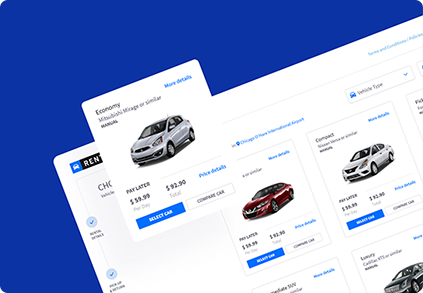The image depicts a screenshot of a car rental website, presented at an angle of approximately 15 to 20 degrees, tilted towards the lower left. The backdrop is a solid blue, creating a stark contrast with the highlighted section. The main section of the website is displayed on a white background, featuring the text "Economy Mitsubishi Mirage or similar." 

To the right, a blue hyperlink labeled "More Details" is prominently featured. Below this, there is a silver Mitsubishi Mirage image followed by the rental pricing information which states, "Pay Later $59.99 per day, $92.90 total." Further to the right, another blue hyperlink titled "Price Details" is visible. Directly underneath these links, on the left side, a blue button with white lettering invites users to "Select Car," accompanied by a white button with black lettering that says "Compare Car."

The image also shows preview snippets of other vehicle options available on the website. Adjacent to the Mitsubishi Mirage is a red Toyota Camry, followed by a silver Nissan Versa, indicating more car choices. Slightly obscured, there are additional categories including "SUV" and "Luxury," with the latter showing a dark green Cadillac XTS or similar.

The overall appearance and elements of the interface suggest that it is from a car rental site, identified by a blue icon featuring a white car and the word "Rent" in white against a black background.